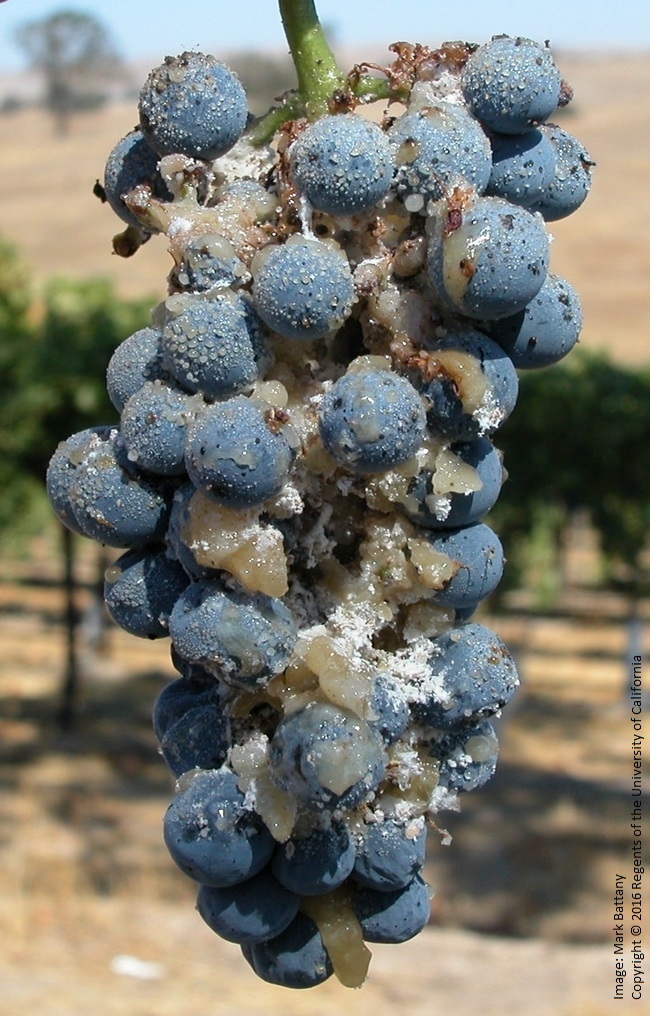The image portrays a cluster of light blue berries, each perfectly spherical in shape, hanging near a rustic wooden fence. A thin layer of frost delicately dusts the scene, indicating a chilly environment. The berries might be vineyard berries, although their exact type isn't clearly identifiable. The softly frosted surroundings add a serene, almost magical quality to the composition.